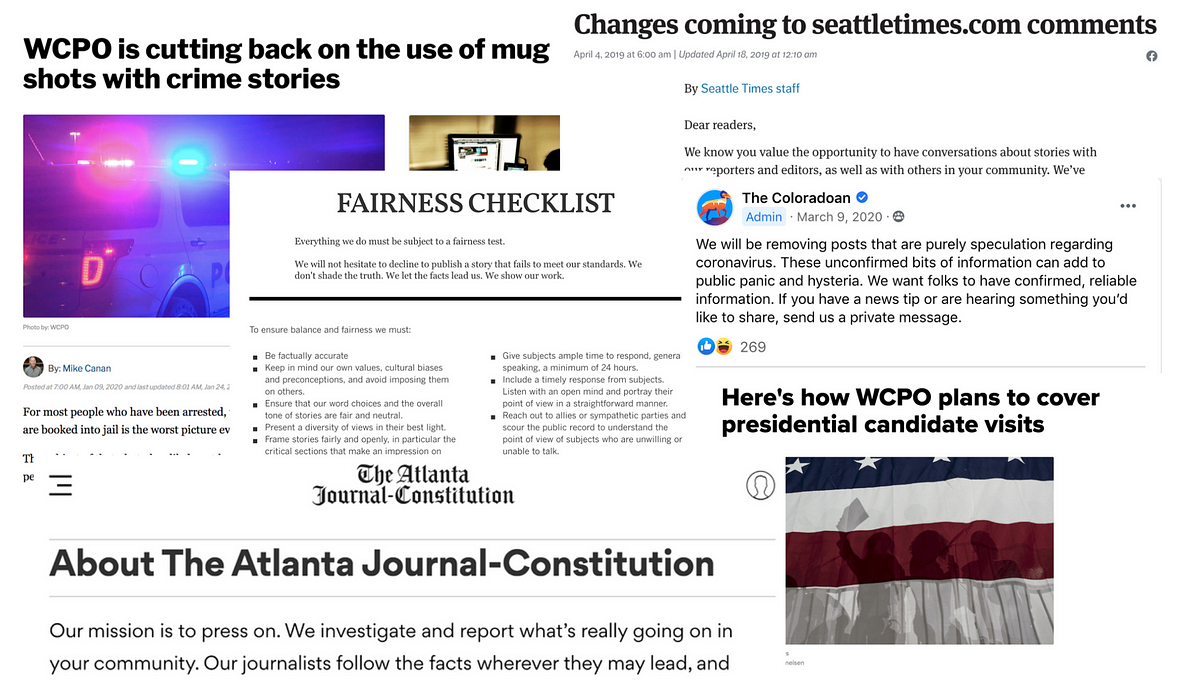The screen capture displays a desktop web page from a news organization, densely populated with bold black headlines. In the upper left corner, the news headline reads, "WCPO is cutting back on the use of mug shots with crime stories," accompanied by an image of blue and red flashing police lights atop a white police car. In the upper right corner, another headline announces, "Changes coming to seattletimes.com comments." Centrally located is the headline text "fairness checklist." On the lower right side of the screen, there is a partial view of the American flag displaying blue, white, and red stripes with stars prominently featured on the blue stripe.